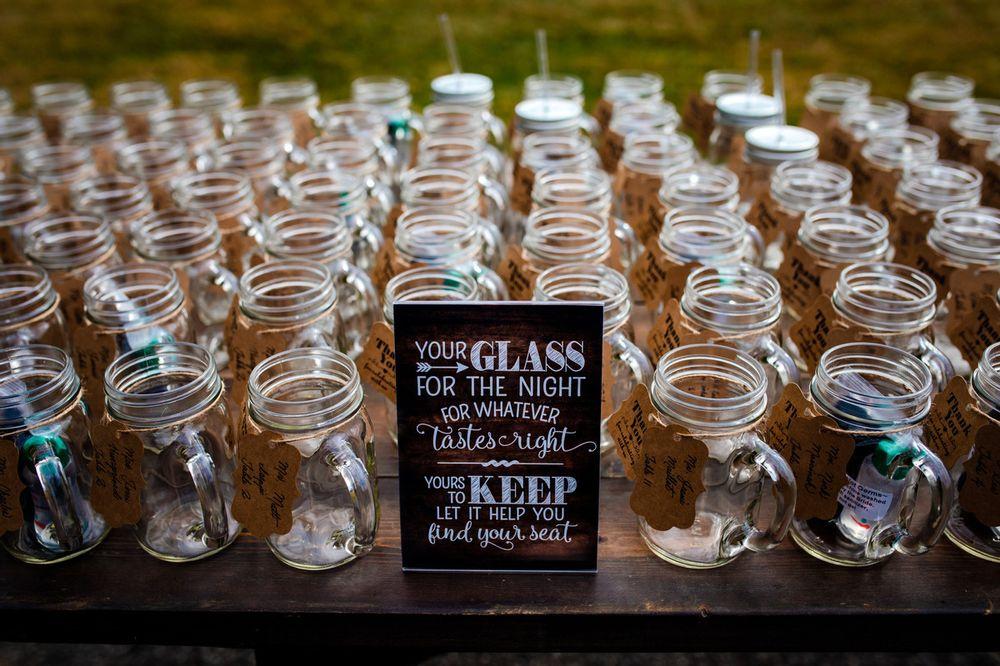The photograph captures an event setup featuring a wooden table lined with approximately a hundred mason jar-style drinking glasses, each jar sporting a handle. These clear glass jars, typically used for canning, are repurposed here as drinking glasses, some adorned with screw-on lids and straws. Each jar is labeled with a brown kraft paper tag that says "thank you," suggesting they are wedding or party favors. Located prominently in the center of the image is a blackboard-style poster with artistic, hipster-style lettering that reads: "Your glass for the night, for whatever tastes right. Yours to keep, let it help you find your seat." The jars at the front of the image are more in focus, with a subtle brown hue contrasting against the clear glass, creating a visually appealing, warm-toned display fitting for a communal celebration.